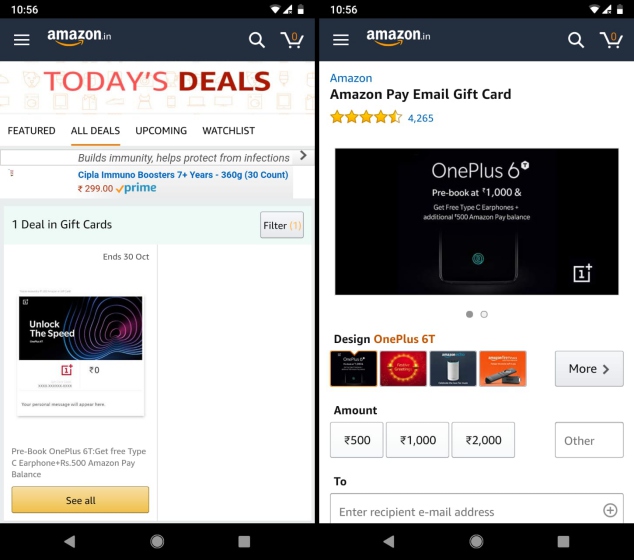The image consists of two side-by-side screenshots taken from an Android phone, both of which are screenshots from the Amazon shopping app. The Amazon logo is visible in the top left-hand corner of each screenshot, indicating the source. The screenshots depict the user in the process of purchasing an Amazon Pay email gift card. 

The right screenshot shows the selection screen for the gift card design, with four different design options displayed. The currency is foreign, although specific amounts like 500, 1000, and 2000 are clearly shown. The screen also includes a field for entering the recipient's email address.

The left screenshot highlights a section for viewing deals, with one specific deal for gift cards that expires on October 30th. The time displayed in the status bar at the top of both screenshots is consistently 10:56.